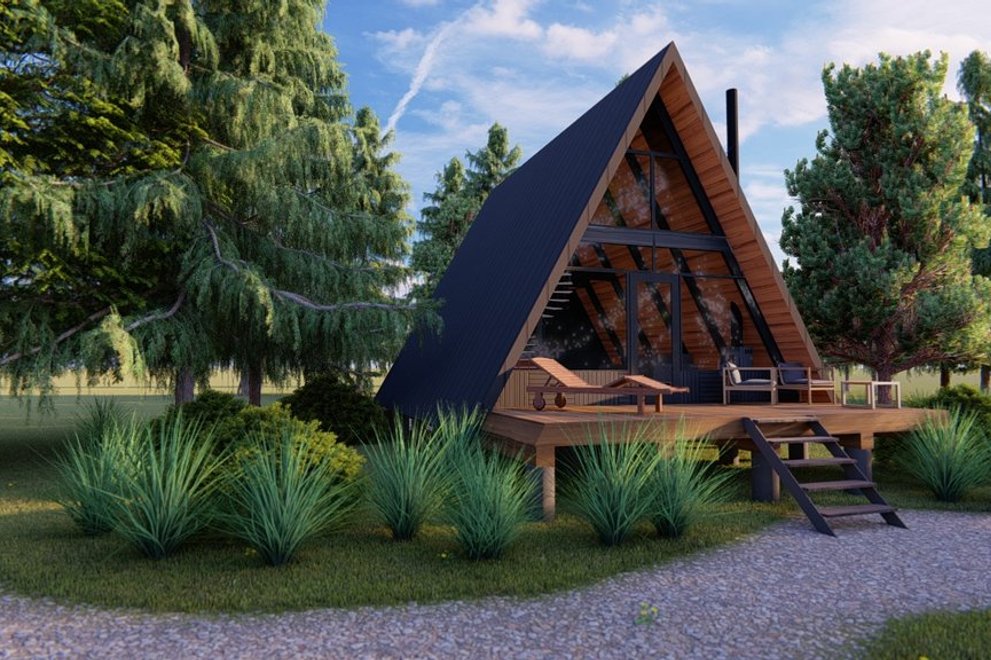The image depicts an architecturally designed A-frame house set against a lush, green landscape featuring evergreen pine trees and spiky shrubs. The house is triangular in shape, predominantly constructed of wood stained in an orange cedar color, and features a striking black trim and roof. The entire front facade is glass, including large triangle-shaped windows and a door. A deck at the front hosts multiple chairs, accessible via black stairs leading down to a gravel walkway that curves through the yard. The setting appears digital, likely an architectural rendering, with realistic elements such as a bright blue sky dotted with fluffy white clouds. The foreground features native grasses, adding to the picturesque and serene environment, further suggesting the house could be a holiday cabin or tiny home.